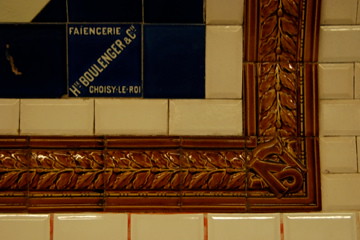The image depicts a section of a wall adorned with off-white beige tiles separated by red grout lines. A significant feature of the wall is a detailed brown wooden frame, situated in the lower right corner. This frame features an intricate ivy-like pattern carved into its border. Inside the frame, the central area consists of white rectangular tiles, further enclosed by a set of black tiles. On these black tiles, white text is visible, although not entirely clear, it includes the name "H. Bollinger" and additional characters that might read "FAIENCERIE H. Bollinger & Cie, CHOISY-LE-ROI." This could indicate the artist or the manufacturer. The setting suggests that this could be the wall of a bathroom, possibly in a business, restaurant, or even a home.